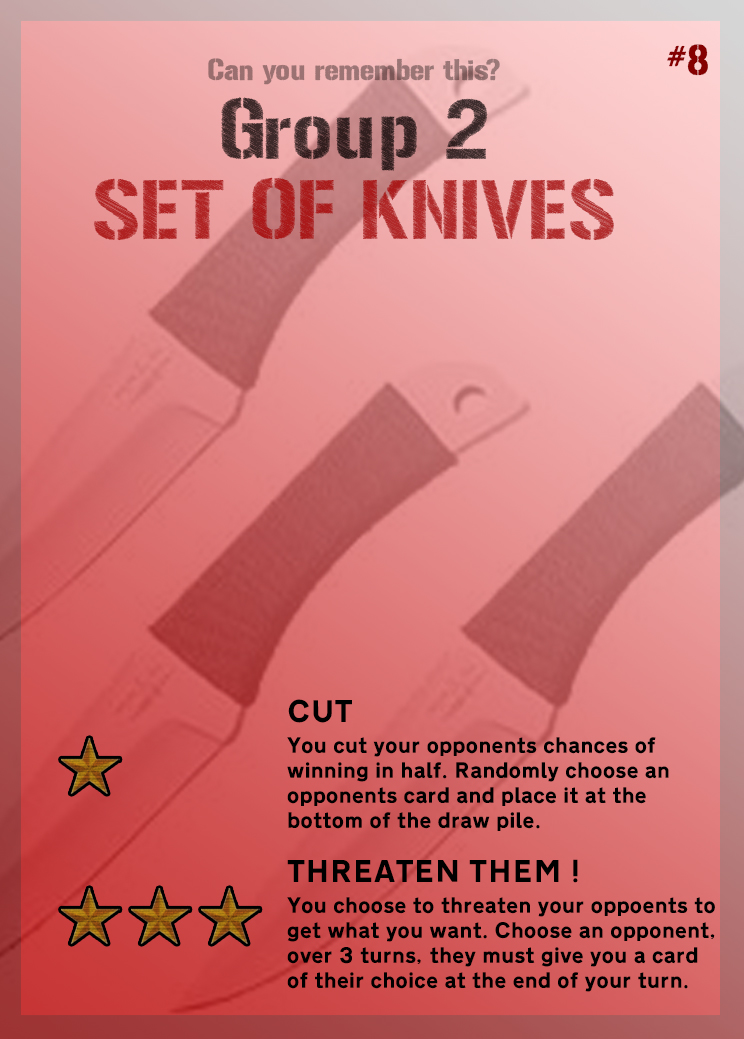The image is a card from a game designed as an infographic. At the top, it features a striking pink background that transitions to a red bottom, encased in a subtle gray border. In the upper right corner, there is a prominently displayed hashtag sign followed by the number 8 (#8). Below this, a central heading reads "Can you remember this" in black text, with "group 2" also in black lettering and "set of knives" in bold red letters. The background showcases three faded chef's knives, each with grip tape around the handle and a silver blade, providing a thematic visual element. 

The card includes two main sections of instructions. The first instruction, prefixed by a single yellow star, reads "Cut: You cut your opponent's chances of winning in half. Randomly choose an opponent's card and place it at the bottom of the draw pile." The second instruction, which appears next to three yellow stars and ends with "Threaten them!" in an exclamatory tone, states: "You choose to threaten your opponent to get what you want. Choose an opponent over three turns. They must give you a card of their choice at the end of your turn." This detailed card appears to be part of a strategic card game, enhancing its interactive gameplay by offering tactical maneuvers.